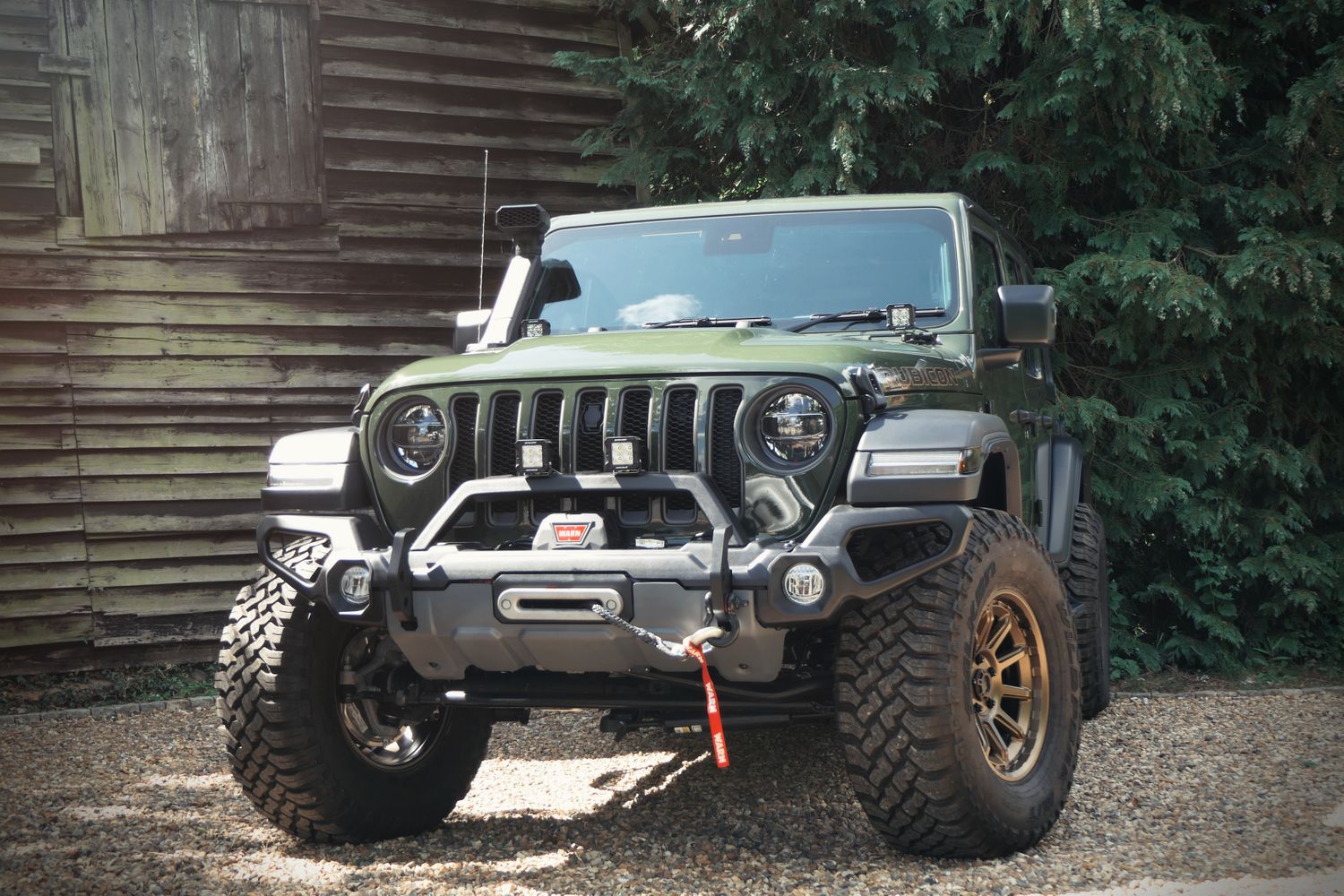This photo captures the front view of a heavily-customized dark forest green Jeep Wrangler Rubicon, also known as a custom Storm 53. The imposing vehicle is parked on a gravel area in front of an old wooden barn or shed, with a cedar or pine tree visible behind it. Distinctive features include a front Venator bumper outfitted with a large winch and additional spotlights on the grill, emphasizing its rugged, off-road readiness. The vehicle is equipped with oversized mud tires mounted on large aluminum rims, further accommodated by extended wheel wells. Prominent round headlights are complemented by extra floodlights near the windshield. The Jeep also features a snorkel, hinting at its capability for water fording.